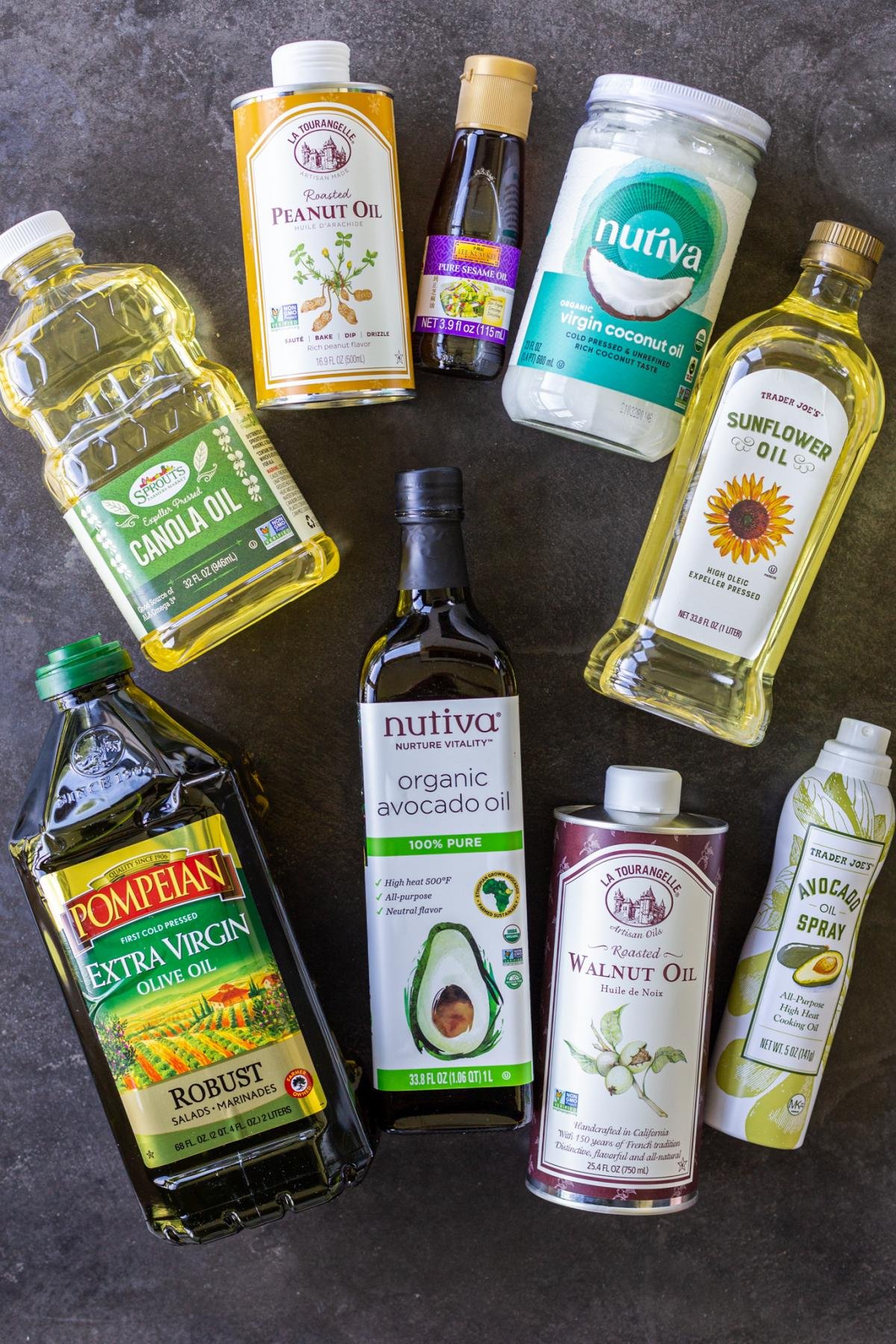The image depicts a variety of cooking oil bottles and cans meticulously arranged on a dark stone countertop. The oils are set in two curved rows, with four items on the top row and four on the bottom. From left to right on the top row, the collection includes a clear plastic bottle of Sprouts canola oil with a green label, a metallic can of peanut oil featuring an orange and white label with peanuts, a sesame oil in a dark glass bottle adorned with a purple label and a gold cap, and a Nutiva organic virgin coconut oil jar with a white label and blue accents. To the far right, completing the upper row, is a Trader Joe's sunflower oil in a clear glass bottle with a white label and a vivid yellow sunflower image.

The bottom row starts with a Pompeian extra virgin olive oil robust variety in a dark green plastic bottle with a familiar branding, followed by a Nutiva organic avocado oil in a white bottle with an avocado graphic. Next, there is a roasted walnut oil that mimics the look of an old metal paint can, displaying a white label with green plant imagery. The row concludes with a Trader Joe’s avocado oil spray bottle that resembles a sunscreen spray, decorated with green leaves and an avocado illustration. The assortment reveals a range of brands, including Nutiva, Le Tourangel, Sprouts, and Trader Joe’s, each with distinct packaging ranging from clear plastic to metal cans, capturing the vibrant hues of yellows and greens within the oils.